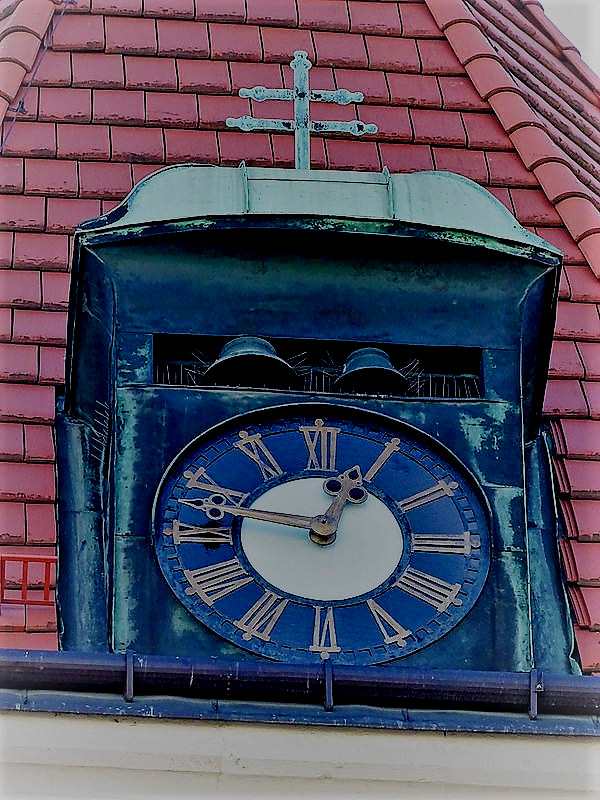This detailed descriptive caption combines all the shared and repeated elements from the given voice captions:

This vibrant color photograph captures an ornate clock mounted on a steeple-like building. The clock features a circular black face with a white center and large gold hands with spade-like tips. The numbers are in Roman numerals, colored in a goldish-brown hue. The clock, displaying the time as 12:53, is surmounted by a metal structure with a double cross at the top. Above the clock face, a large rectangular housing contains two prominent black metal bells. The clock and bells are set against a background of red terracotta tiles, arranged in a conical shape with round angles and square sections on the front and sides of the roof. The photo, taken during the day, captures the rich colors and intricate details, making it appear almost like a watercolor painting.